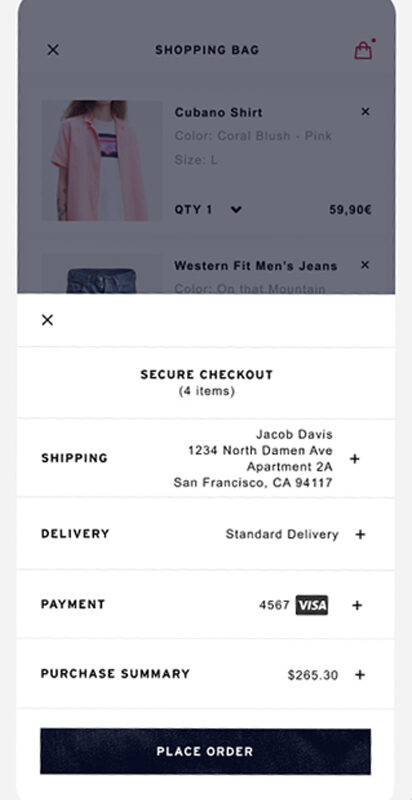This is a screenshot of a cell phone displaying an online shopping page during the secure checkout process. The main focus is a pop-up box, which appears against an opaque dark grey overlay that partially obscures the site background. Despite this, the background remains somewhat visible.

In the background, at the top center of the image, the text "Shopping Bag" is prominently displayed. To the far left, an "X" icon provides an option to close the shopping bag view, while a handbag logo is situated all the way to the right. Below this, there is a thumbnail image of a woman modeling a t-shirt and a pink open button-up Cuban shirt. The item's details reveal that it is a large-sized Cubano shirt, priced at €59.99, with a quantity of one in the bag.

The pop-up box in the foreground has a white background with black text. In the top left corner, another "X" icon allows for closing the checkout window. The header "Secure Checkout" is prominently displayed, followed by the indication "(4 items)" in brackets.

A thin grey line separates different sections within the pop-up. The first block labeled "Shipping" appears on the left, with the shipping address right-justified on the right: Jacob Davies, 1234 North Damon Avenue, Apartment 2A, San Francisco, CA 94117.

Another thin line divides this from the next section, "Delivery," where the standard delivery option is selected. A subsequent line separates this from the "Payment" section, showing the last four digits of the Visa card, 4567. Another dividing line leads to the final section, "Purchase Summary," which totals $265.30.

At the bottom center of the pop-up, a large rectangular black button with the text "Place Order" in white stands ready for the final confirmation.